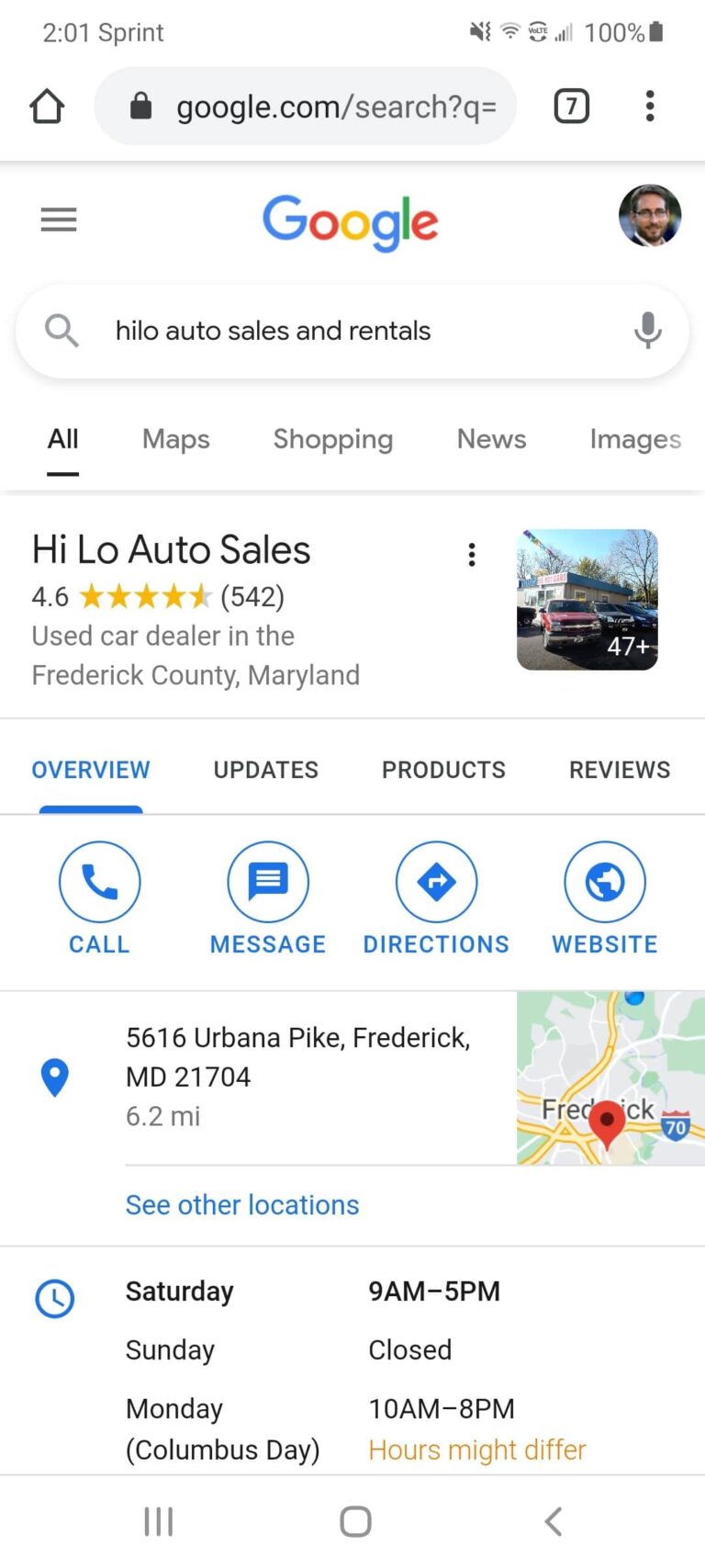Here is your revised and detailed caption:

---

The image depicts a screenshot of a cell phone displaying a Google search for "Hilo Auto Sales and Rentals." The status bar at the top shows the time as 2:01 PM, the carrier as Sprint, with the device on vibrate mode, full Wi-Fi signal strength, and "VoLTE" capability. The battery is fully charged at 100%.

Below the status bar, the Google search interface is visible. The search URL reads "google.com/search." A profile picture of a man with dark hair is displayed beside the "Google" logo in its signature colors. 

The search query entered is "Hilo Auto Sales and Rentals," bringing up the search results tab labeled "All," highlighted with a blue underline. Other tabs available are "Maps," "Shopping," "News," and "Images," all in black text.

The first search result shows "Hilo Auto Sales" with a rating of 4.6 stars based on 542 reviews, categorized as a used car dealer in Frederick County, Maryland. The details are organized under tabs "Overview," "Updates," "Products," and "Reviews," with "Overview" currently selected and highlighted in blue.

A row of action buttons is displayed below, offering options to "Call," "Message," "Directions," and "Website." Below this, the address "5616 Urbana Pike, Frederick, MD, 21704, 6.2 miles away" is provided, along with a small map thumbnail.

---

This version condenses and organizes the information to make the caption more comprehensive and reader-friendly.